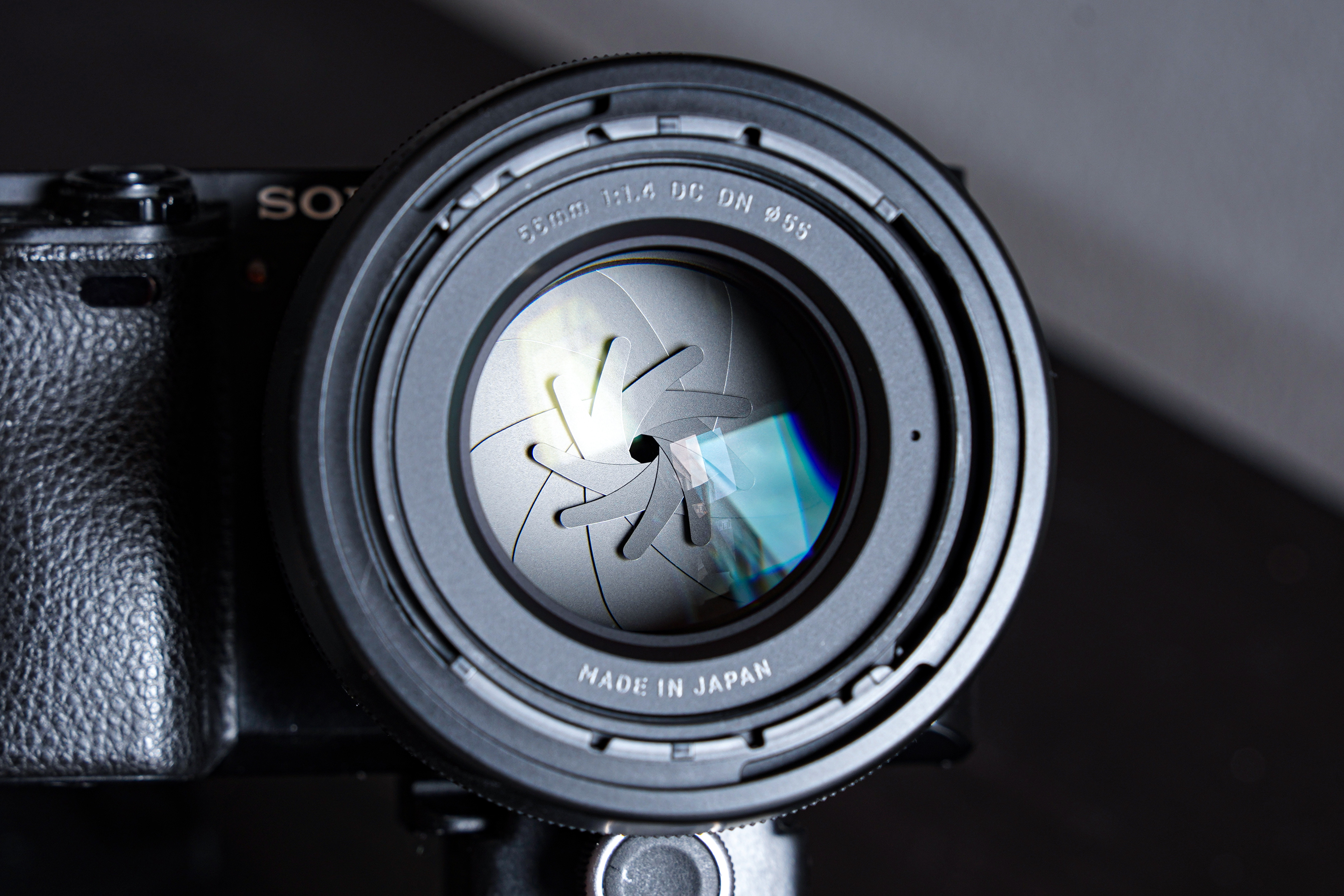A detailed close-up image of a Sony camera lens is the primary focus, prominently featuring a 55mm f/1.6 DC DN lens, marked "Made in Japan." The lens showcases an intricate design with visible glass elements and is slightly indented, revealing mechanics that allow for manual focus adjustments. The surrounding ring has an 'E' marking visible at both the top and bottom positions. The lens appears to be in the midst of capturing a photo, with the shutter partially closed. To the left of the lens, part of the camera body, wrapped in a black leather casing that seems to have a textured, snake-skin appearance, is visible, along with a flash button and the partially readable letters "SO," indicating it's a Sony camera. The camera is mounted on a tripod with a black knob for adjustments. The background adds contrast, appearing as a blurry mix of black and gray, highlighting the sharp details of the lens and the reflections from the lighting.